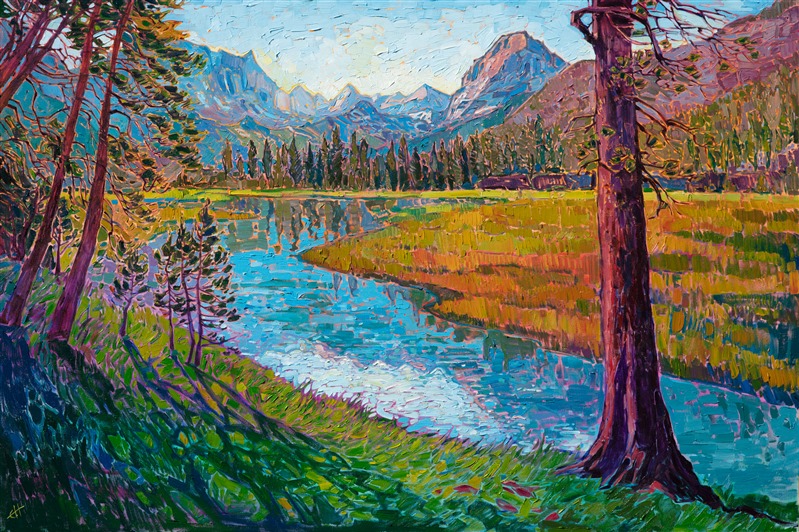This image is a detailed neo-impressionist painting depicting a vibrant valley scene. The foreground features a lively stream that originates from the lower right corner, meandering towards the center and then curving back to the left, eventually disappearing into the distance. The brush strokes are quick and small, applied in bold, thick dabs to create a textured, vibrant effect. 

On the right side near the stream's origin, there's a prominent tree with a purple and brown trunk extending upward. To the left of the stream, a variety of tree trunks exhibit shades of purple-reddish tones. The grassy areas on both sides of the stream are painted in an impressionistic style, with a mix of greens, yellows, and reds, interspersed with blues and purples.

In the background, tall mountains rise on both sides and slightly in the center, their peaks touching a sky painted in shades of blue and white. The forest at the base of these mountains has a reflective quality, mirrored subtly in the stream's water. Adding to the overall striking appearance, there's a pervasive pink tinge replacing where shadows might typically be black, giving the scene a surreal, luminous quality. In the far distance, low brown shapes suggest possible farmstead buildings, blending seamlessly into the landscape.